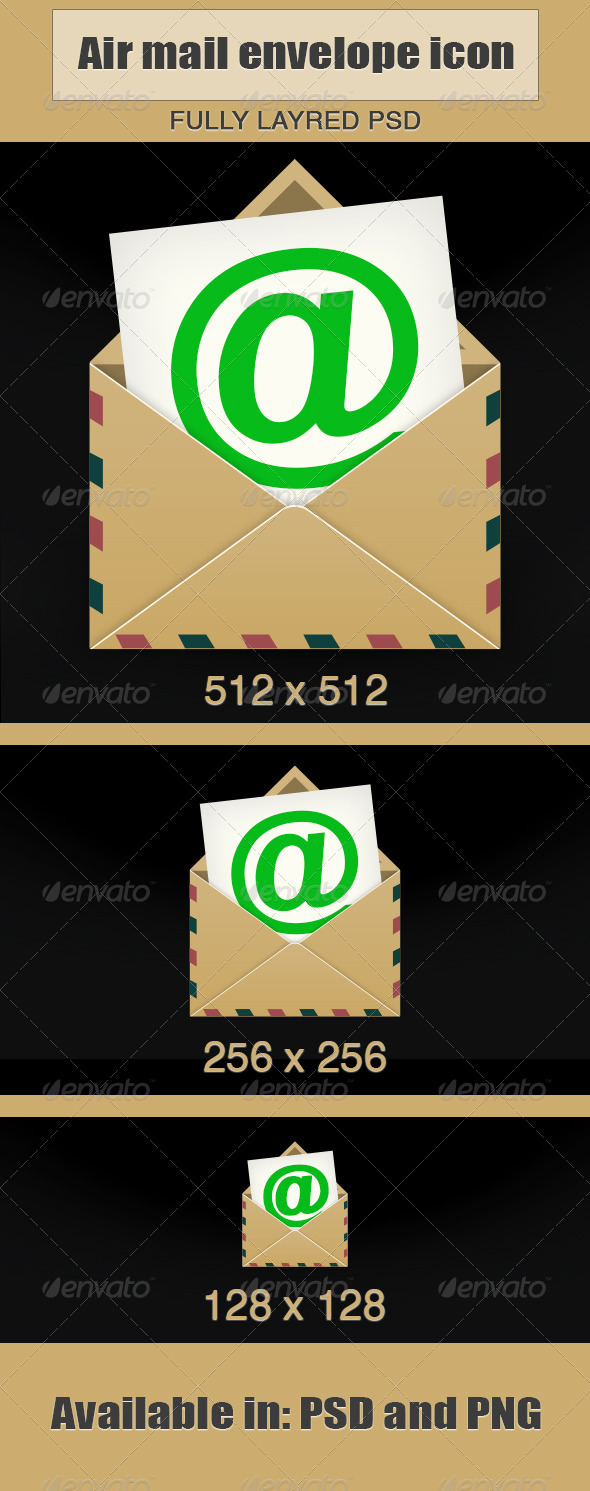This image showcases a digital drawing advertising the availability of an airmail envelope icon in various sizes and formats. At the top, against a cream background, the black text reads "Air Mail Envelope Icon." Below this, on a brown background, another line of black text states "Fully Layered PSD." Centrally displayed against a black background is the main icon, featuring a brown envelope with dashed red, brown, and dark green lines along its edges. The envelope is open on the backside, revealing a white piece of paper with a prominent dark green "@" symbol. Below the icon, text indicates different size options: "512x512," "256x256," and "128x128." At the bottom, the text notes that these icons are "available in PSD and PNG” formats. This image appears to be a stock image potentially from a company like Envato, which often leaves watermarks and might include a small logo resembling a flower or a leaf. The overall arrangement is vertically stacked, with each element centered within its respective section. The colors predominantly featured are brown, tan, black, green, and white, contributing to a cohesive and organized visual presentation.